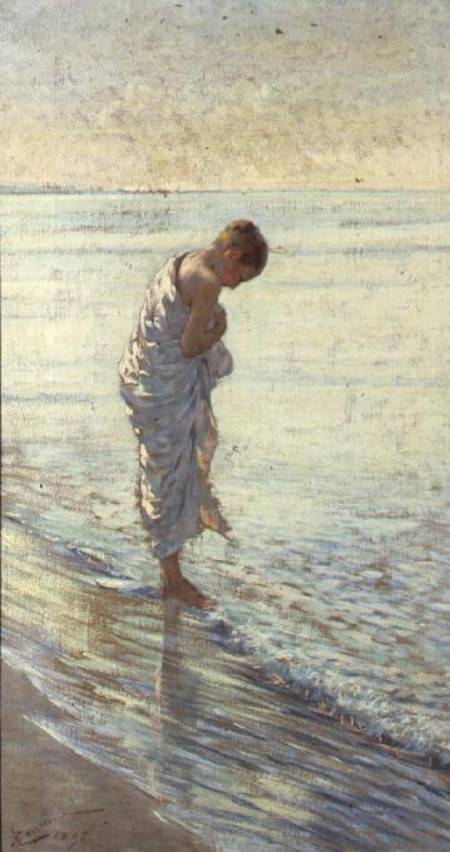The painting, set on a long, aged canvas, depicts a lone figure standing at the edge of a shoreline, possibly a river or a sea. The figure is draped in a white, sheet-like garment, suggesting nudity underneath, with the upper back, right shoulder, and arms exposed. The figure's head is bowed, and short hair is tied back, indicating a contemplative stance as they look down into the water. Their feet are poised at the water’s edge, with gentle waves lapping at their toes and reflecting their image.

The scene is rendered in a harmonious color palette of beige, light blues, and whites, creating a serene and unified composition. The water, characterized by shades of blue and white, stretches into the horizon, where no landmass is visible, further emphasizing the solitary nature of the scene. In the lower left corner of the painting, there is a signature that includes at least the initial 'K' and the date 1895, suggesting the artwork's historical value.